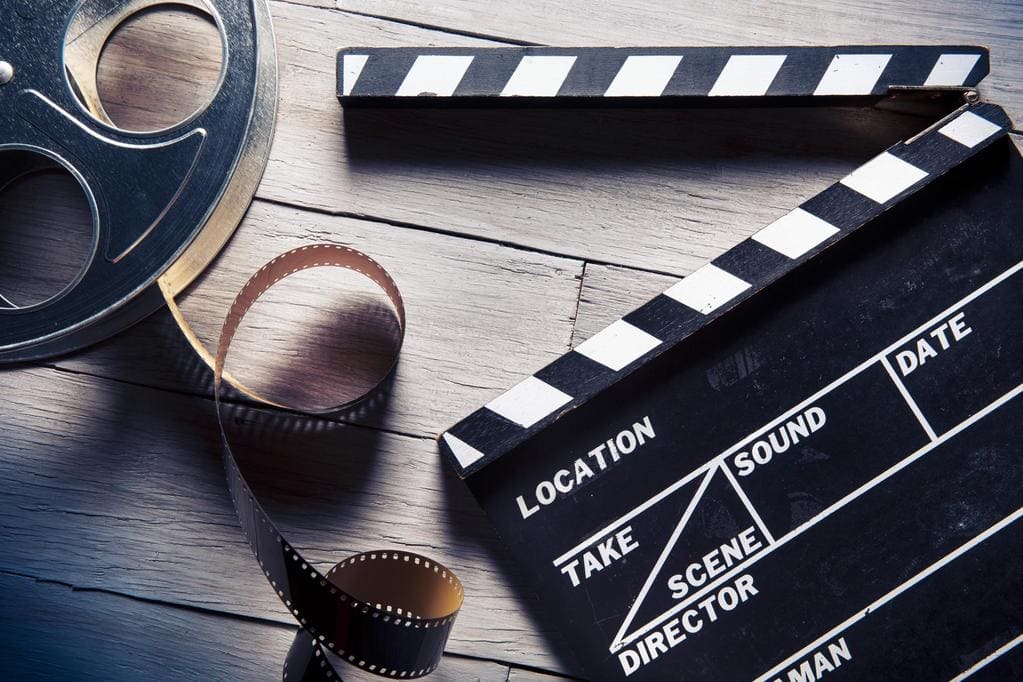The image is an overhead photograph capturing a scene on a gray wooden table. On the table to the upper left, there's a metallic film reel with a small amount of brownish celluloid film trailing diagonally down towards the bottom left of the image. On the right side of the photo, a classic black-and-white clapperboard, often used on film sets to mark scenes with a “clap” sound, is prominently positioned. The clapperboard, identified by its wooden boards, displays various labeled sections including "Scene," "Take," "Sound," "Date," "Director," and "Location." The colors visible in the photograph include shades of gold, black, white, gray, and light yellow.